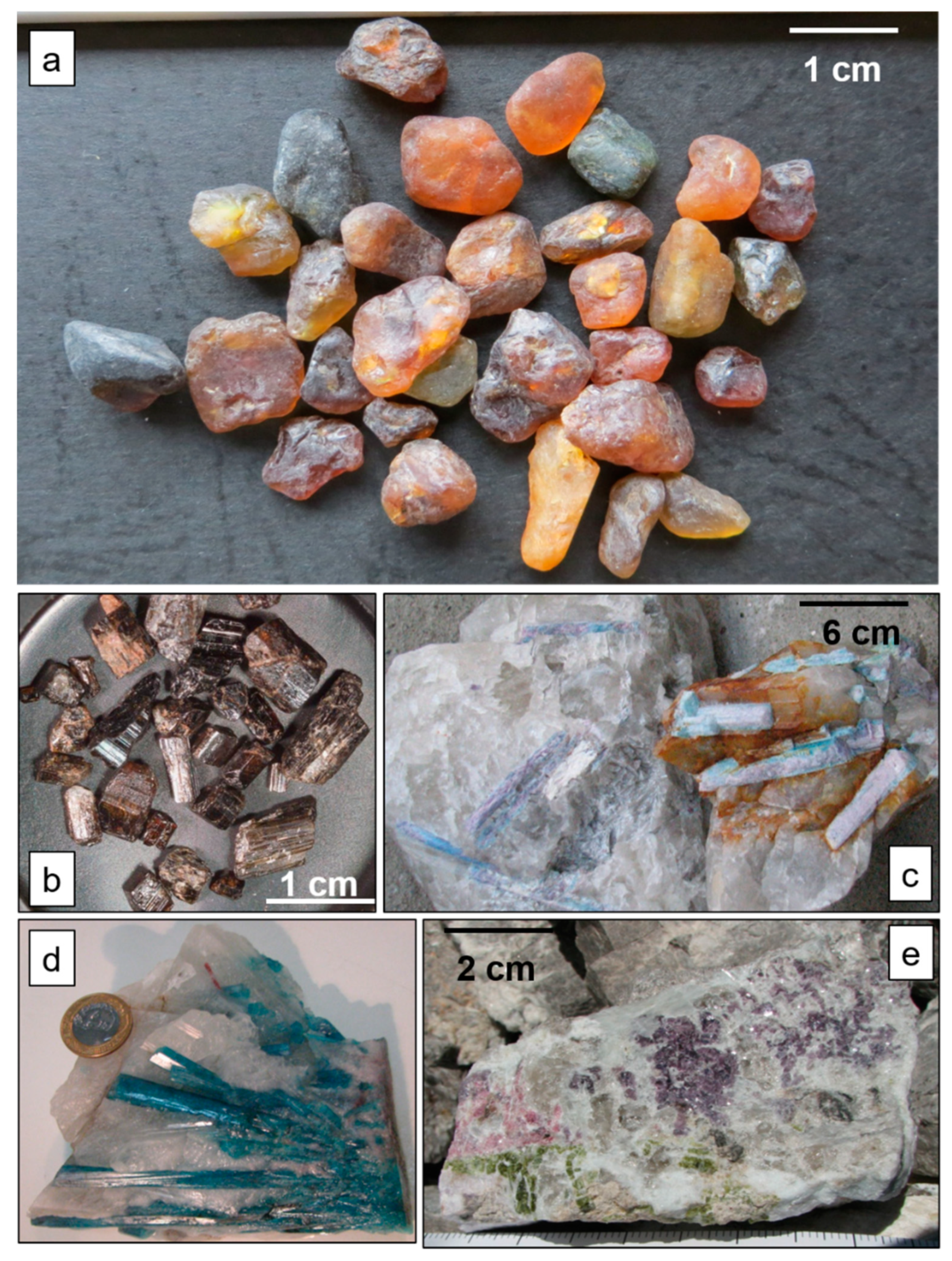The image is a collage of five detailed photographs of various stones and minerals, arranged in labeled sections A through E, each showcasing different colors and sizes with scales provided for context. Section A, occupying the largest portion at the top, presents an array of irregularly shaped stones in hues of gray, orange, pink, and yellow, each approximately one centimeter in size. Below, Section B features one-centimeter brown rocks or crystals with a shiny, semi-transparent quality. Section C, measuring six centimeters, displays larger pieces with gray stones and hints of brown. In Section D, a clear stone with turquoise striations is shown alongside a coin for scale, although its exact size is not specified. Lastly, Section E contains a clear rock about two centimeters in size with rose and purple tones, and possibly hints of green embedded within it. All sections are set against plain backgrounds to emphasize the stones' natural beauty and detail.